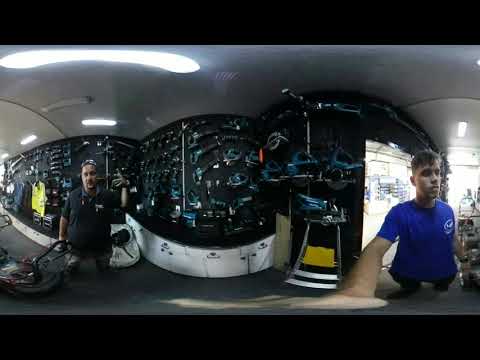Two men are inside what appears to be a workshop or a drone studio. The man on the left is wearing a black short-sleeved work shirt and jeans that seem slightly ripped. He is holding something up in his gloved left hand. The man on the right wears a blue t-shirt with a symbol on it and black pants; his right hand rests on an unidentified machine or possibly a lawn mower-like device. Both men have their bodies facing towards the viewer although the man in the blue shirt looks left, and the man in the black shirt looks more to the right.

The background is characterized by a black wall adorned with various tools and equipment, some of which might be related to drone mechanics as suggested by the numerous parts on display. The floor is grey, and a fluorescent light fixture hangs from the low ceiling, casting a glare. Additionally, a yellow jacket can be seen hanging further to the left. A distorted perspective makes the limbs of the man on the right appear unusually proportioned, particularly his forearm. The photograph is dark, emphasizing the workshop's clutter and the industrial ambiance.